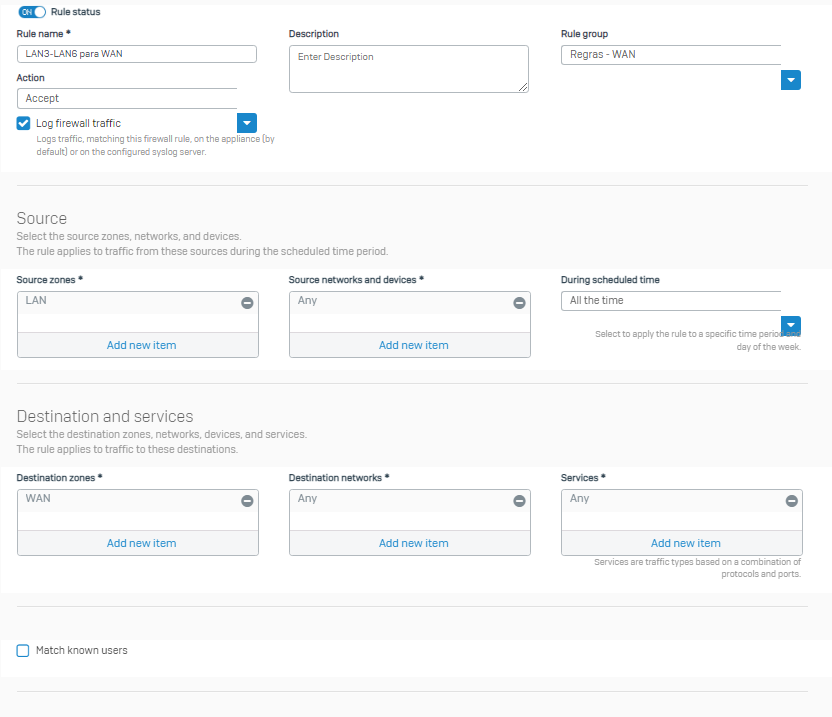The image displays a detailed user interface of a computer screen, showcasing a complex network rule configuration panel. 

At the top left corner, there's a blue toggle switched on, indicating the "Rule Status." Directly beneath it, there's a labeled text box for the "Rule Name," followed by another text box for "Action." Below these sections, there's a checkbox labeled "Log Firewall Traffic," which is currently checked.

To the right, there's a text box for "Description," with a prompt inside that reads "Enter description." Adjacent to it is a labeled text box for the "Rule Group." A horizontal line separates these sections from the following content.

Underneath the line, there's a section titled "Source" where users can add "Source Zones," "Source Networks," and "Devices." Additionally, this section allows configurations for "During Scheduled Time."

Another horizontal line appears, separating the "Source" section from the "Destination and Services" section. Here, users can select the "Destination Zones," "Destination Networks," "Devices," and "Services" to which the rule applies. Guidance text specifies that the rule impacts traffic directed towards these destinations.

In the bottom left corner, there's an empty blue checkbox labeled "Match Known Users."